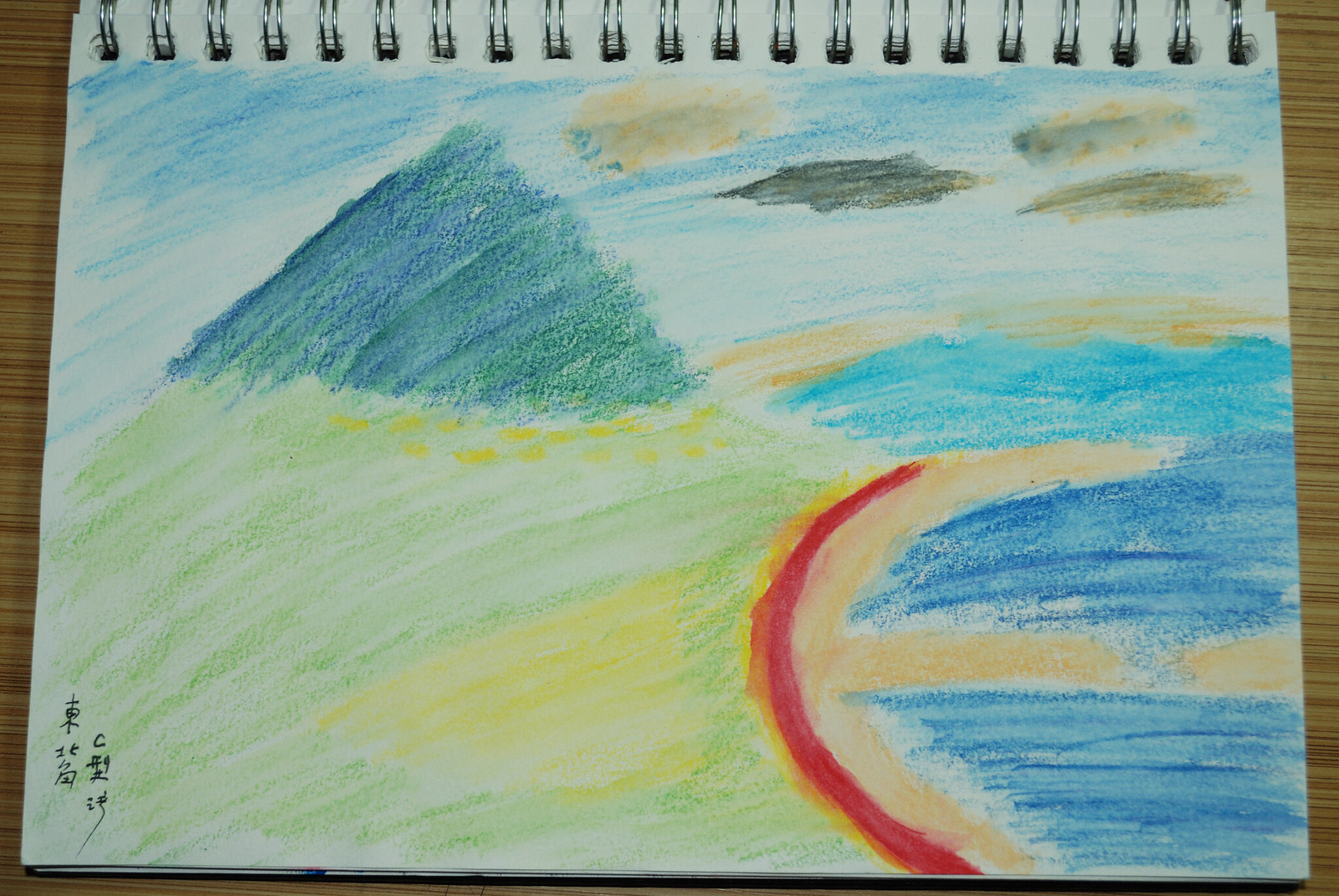This is a detailed colored pencil drawing on plain white paper, captured in a photograph. The artwork, housed within a spiral-bound sketchbook, prominently features a mountain rendered in shades of blue and green, with a backdrop of a blue sky. Dark gray clouds dot the sky, partially obscuring a yellow sun. Below the mountain, a landscape of yellow and green grassy fields transitions into a beach area. The beach itself is detailed with tan sand, adorned with a red stripe and a yellow stripe. The ocean waves, depicted in varying shades of blue, gently lap against the sandy shore. In the bottom corner of the drawing, black characters resembling Japanese or Chinese script add an element of mystique and cultural depth to the scene. At the top of the image, decorative spirals contribute to the artistic flair of this handmade piece.